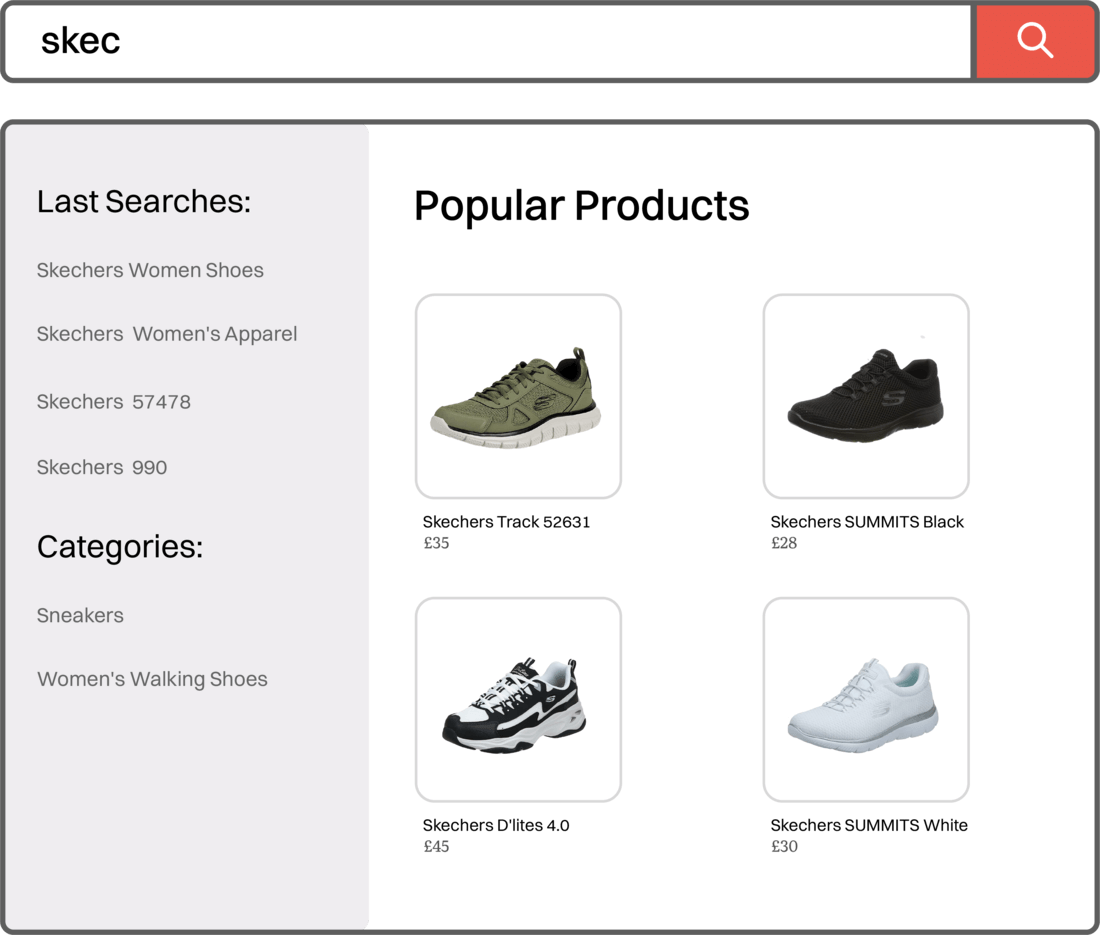This image is a screenshot from an unspecified source, featuring a user interface with a search function at the top. The search bar contains the typed query "SKEC." To the far right of this bar, there is a red icon with a white magnifying glass, indicating the search button.

Below the search bar, a vertical menu lists various search suggestions and categories: 
- Last Searches
- Sketchers
- SKECHERS
- Women's Shoes
- Sketchers Women's Apparel
- Sketchers 57478
- Sketchers 990
- Categories
   - Sneakers
   - Women's Walking Shoes

To the right of this menu, the section titled "Popular Products" is displayed. This section showcases several items:
- A photograph of a gray sneaker with gray laces, a white sole, and an "S" logo on the side. The description reads "Sketchers Track 52631, £35."
- An image of a black sneaker with a black "S" on the side, labeled "Sketchers Summits Black, £28."
- Another image depicts a black and white sneaker with white laces, labeled "Sketchers D'Lites 4.0, £45."
- Finally, an image of a white sneaker is shown with the description "Sketchers Summits White, £30."

This interface does not contain any human or animal images.